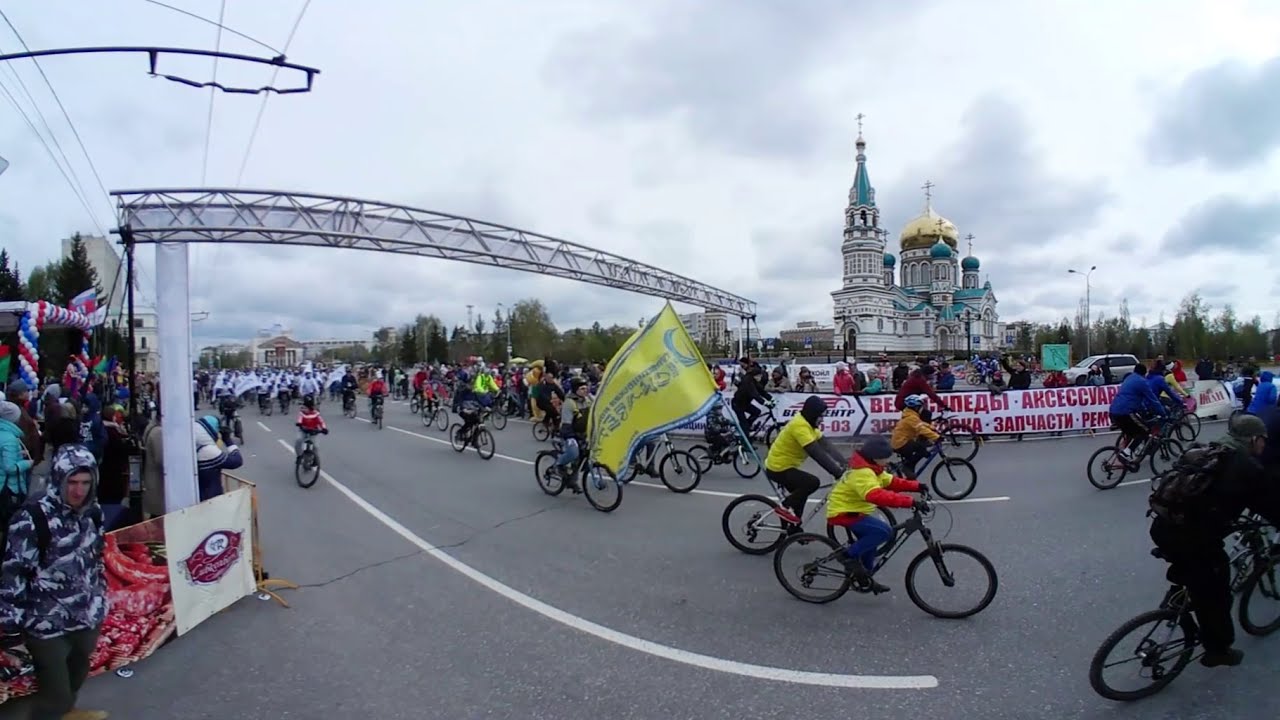The photograph depicts an intense bike race or festival occurring on an overcast, chilly day, as suggested by the bundled-up spectators and participants. A multitude of cyclists, some wearing bright colors, dominate the asphalt road, with one conspicuous rider bearing a large yellow flag from their bike. The scene is bustling with onlookers, some in white raincoats, standing behind railings adorned with banners. A metal frame arching over the road adds to the festive ambiance, hinting at a formal race event. In the background, a grand European or Russian-style cathedral or palace towers, distinguished by its white concrete structure, gold domes, and teal accents. The sky is predominantly gray and cloudy, cultivating a dreary yet vibrant atmosphere. Additional elements such as balloons, barricades, and police presence emphasize the race's significance and the community's engagement.